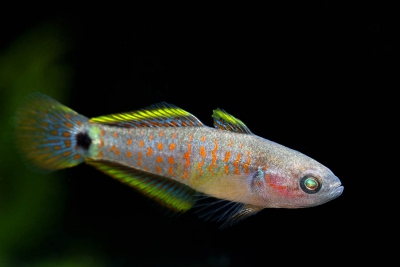The image captures an exquisite exotic fish set against a stark black background, highlighting its vivid features. The fish's body is adorned with vibrant orange spots set against a whitish-gray backdrop, creating a striking contrast. Its eye is a captivating teal color, adding to its allure. The fish has two dorsal fins, each tipped with bright yellow and marked with white and orange patterns beneath. The singular ventral fin also boasts yellow tips. The tail, slightly blurry and distorted in the image, features a distinctive black spot at its base and is accented with yellow tips. The fish's intricate color patterns and the impeccable focus on its vibrant hues make it an exceptionally beautiful specimen.